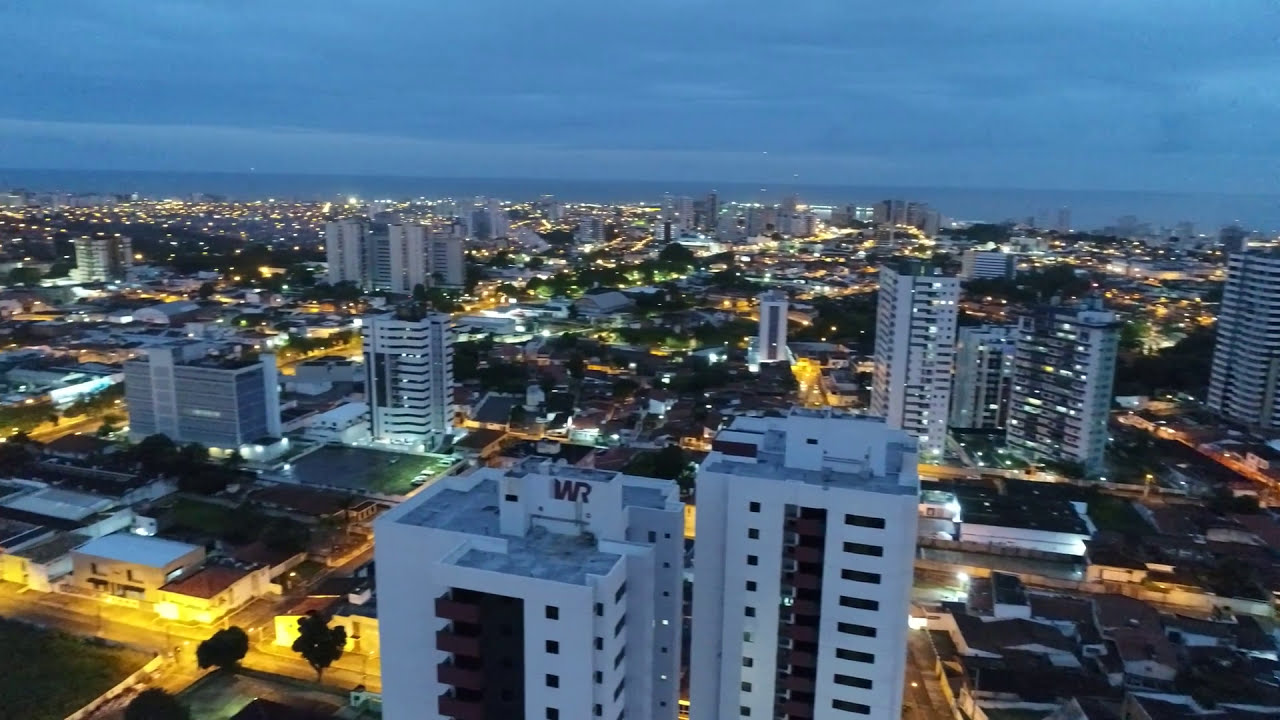This image presents a detailed aerial view of a city during twilight, showcasing a myriad of industrial and residential buildings, including numerous skyscrapers and apartment complexes. The vantage point appears to be from a tall building or aerial perspective, providing a sweeping look over the cityscape. The sky at the top of the horizontally aligned picture is a bluish-gray, filled with layers of clouds. Towards the horizon, the sky transitions to a deeper blue.

In the foreground, at the very bottom, stands a prominent white building with the letters "WR" at its top, possibly a hotel. Adjacent to this building, on the left and right, are similarly tall structures, predominantly colored in white or light gray stone. Scattered among these towering edifices are shorter residential buildings with characteristic brown roofs, interspersed with tree-lined streets.

The city is alive with illumination; numerous lights punctuate the scene, highlighting roads, street lamps, and the steady flow of traffic at ground level. The image captures the intricate network of roads weaving through the city, some lit in yellow hues from street lamps. The distant backdrop hints at a body of water under the night sky, adding depth to the urban landscape. The overall ambiance is one of a bustling metropolis transitioning from day to night, with a vibrant skyline and sparkling lights marking the end of the daily commute.